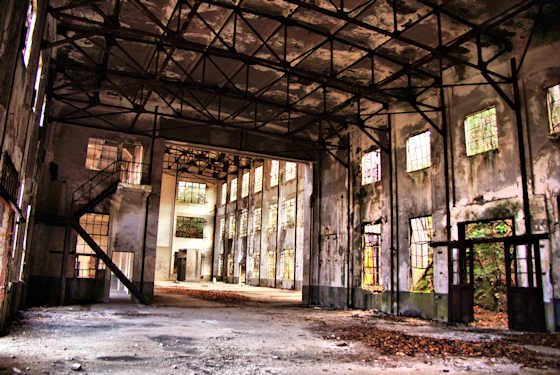This image captures the interior of an abandoned, industrial-style warehouse, taken during the daytime. The concrete structure features tall, black steel beams crisscrossing the high, unfinished ceiling and spanning the walls. The abandoned warehouse, likely two to three stories high, has a deteriorating interior with a dirty, crumbling cement floor littered with rocks, debris, and a pile of brown leaves. Large, square window panes, many with bars but possibly missing glass, line the walls, allowing plenty of natural light to flood the space and illuminating the green trees and forest visible outside. An open exterior door provides easy access inside, while a black staircase on the left leads to the upper floors. The walls of the warehouse exhibit a mix of light and dark gray hues, adding to the overall sense of decay and abandonment.